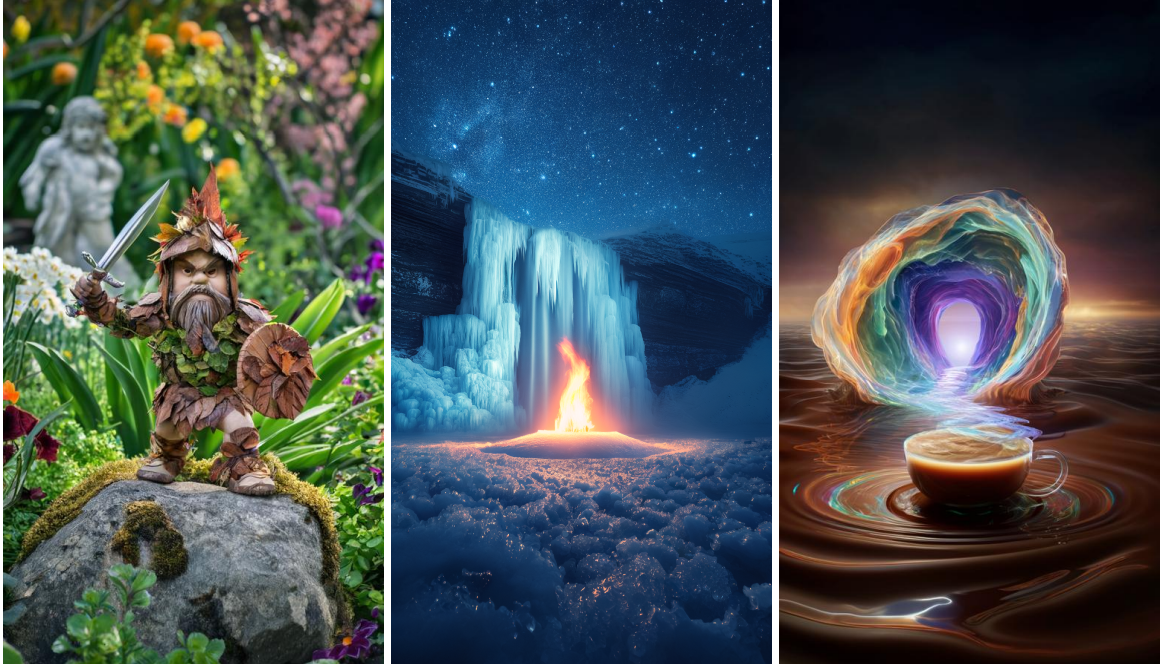This image showcases three distinctly different and captivating pictures arranged from left to right. 

On the left, the first picture features a whimsical garden gnome adorned in a leaf vest and helmet, bravely holding up a sword amidst a vibrant garden scene. The middle image captures a mesmerizing winter landscape, highlighting a frozen waterfall with intricate ice formations cascading from a rock. At the bottom of this scene, an ethereal orange flame flickers, adding a touch of warmth to the frosty wonderland. 

To the right, the third picture transports us to a surreal universe, where a dark tan coffee cup, set in a clear mug, releases a magical swirl of steam. This steam transforms into a colorful tunnel of greens, purples, and golds, creating a fantastical and trippy visual experience. The collective hues of greens, reds, yellows, whites, dark blues, fiery reds, purples, and browns tie these diverse images together, offering a rich and vivid tapestry of scenes and colors.